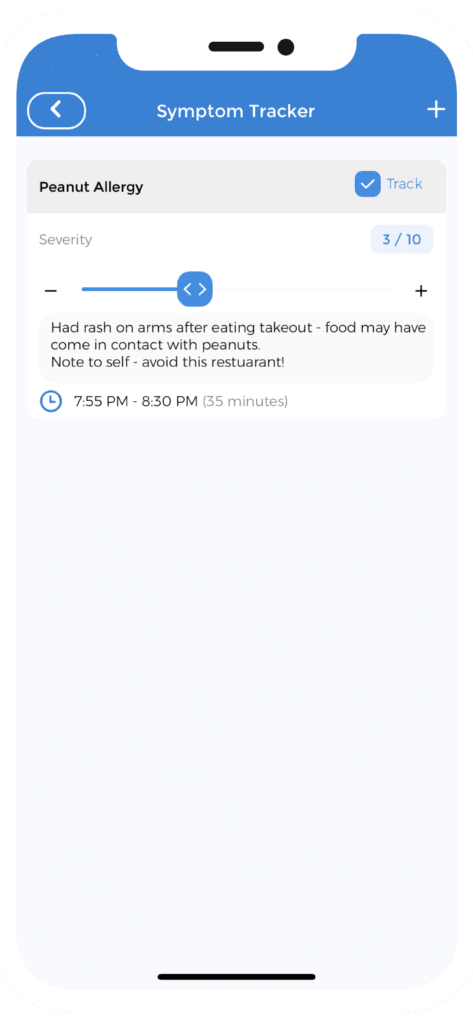This screenshot captures an insightful snapshot from an allergy tracking mobile app.

**At the very top of the screen**, the header bar is blue and prominently features the title "Symptom Tracker." The top-right corner displays a plus sign, presumably for adding new entries, while the top-left corner has a circular icon with a left-pointing arrow, likely for navigating back to a previous screen.

**Just beneath the header**, the screen identifies the specific allergy being tracked with the label "Peanut Allergy." There is a blue check-marked box next to the word "Track," indicating that the user is actively monitoring this allergy.

**The main content area** includes detailed information about a specific allergic incident:
- **Category**: Listed as "Severe."
- **Description**: The user reported experiencing a rash on their arms after consuming takeout food. They suspect the food might have come into contact with peanuts, highlighted by the note "#food may have come in contact with peanuts."
- **Personal Note**: "Note to self: avoid this restaurant," indicating a precaution for future reference.

**A blue clock icon** signifies the duration of the allergic reaction, detailed as occurring from 7:55 PM to 8:30 PM, totaling 35 minutes.

**Under the severity scale**, a segmented bar allows users to rate the intensity of symptoms from 3 to 10. The user has marked this particular incident with the maximum severity level, a 10.

This detailed tracking entry provides a comprehensive overview of the allergic reaction, aiding the user in identifying and managing their peanut allergy more effectively.